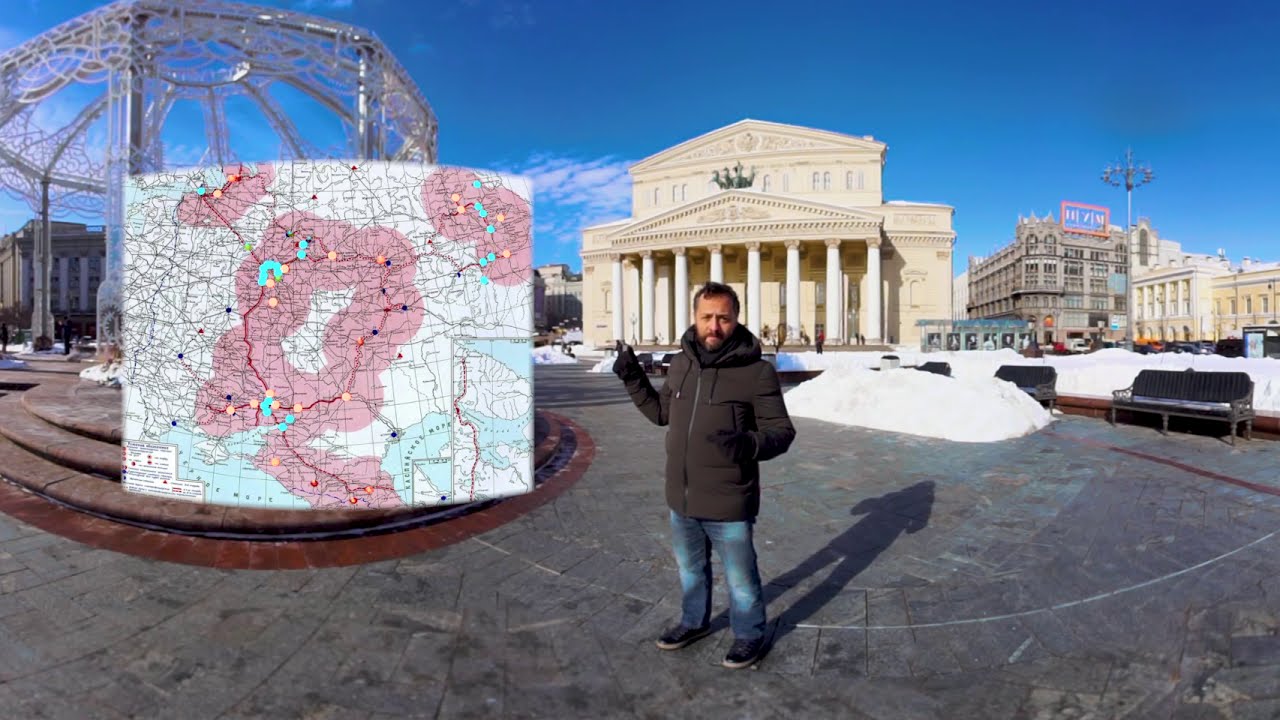The image depicts a bustling city square, likely in Moscow, with the iconic grandeur of a famous theater as a backdrop. Dominating the scene is a large white building with eight or nine imposing pillars, made of white or tan limestone, enhancing the classical architectural aesthetics. Adjacent to this structure is another tall building adorned with a distinctive blue sign edged in orange. A central figure, a man with black hair and olive-colored skin, stands prominently in the foreground wearing a puffy black coat, blue jeans, and black shoes or sneakers. His right hand gestures towards a large exterior map positioned on the left side of the image, seemingly overlaying a gazebo that resembles a delicate crystal or lace framework. The gazebo itself, featuring geodesic-style windows and three brick steps, sits centrally in the round park area surrounded by empty benches, indicating recent snowfall. The man appears to be explaining something, adding a dynamic element to the serene, snow-dusted cityscape.